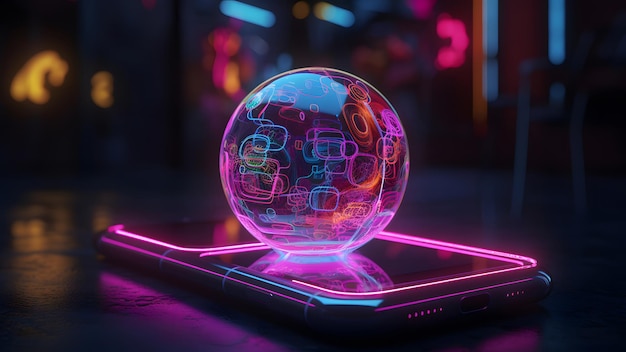The image is a photograph of a futuristic scene featuring a black mobile device, likely a phablet, bordered by a vibrant pink neon glow. Perched atop the device is a transparent glass orb adorned with various multicolored, rounded square shapes in hues of blue, orange, pink, and green. The overall setting is dark and somewhat out of focus, with a background that melds into an abstract blur of colors including yellow, blue, and red, adding to the enigmatic atmosphere. The entire composition gives off an artificial intelligence and cyberpunk vibe, with the intricate details of the neon-bordered device and the glowing, colorful elements within the glass orb drawing the viewer's attention.